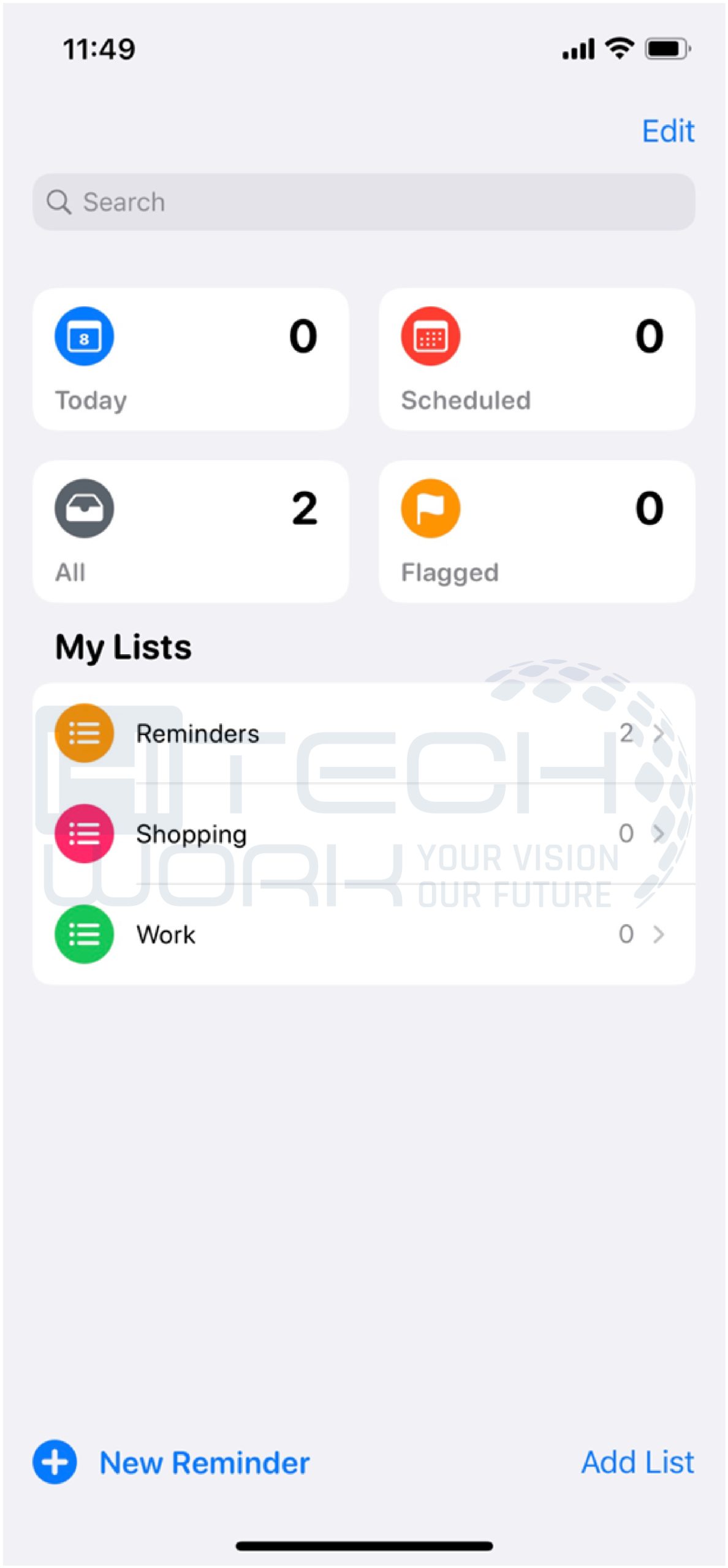The image is a screenshot taken from a mobile phone app. The time displayed in the upper left corner reads 11:49. On the top right are icons showing signal strength, Wi-Fi connectivity, and battery status. Below these icons, aligned to the right, is an "Edit" button in blue. Stretching across the screen is an elongated oval search bar with a magnifying glass icon to the left, and the word "Search" in a grayed-out font.

Beneath the search bar, the interface is divided into four sections, each enclosed within a white rectangle. The sections are labeled "Today" with '0' tasks, "Scheduled" with '0' tasks, "Flagged" with '0' tasks, and "All" with '2' tasks. 

Further down is a section titled "My List" in bold black. This section is divided into three subsections: "Reminders" with '2' tasks, "Shopping" with '0' tasks, and "Work" with '0' tasks. Next to each subsection name is a circle icon with three horizontal lines, color-coded as follows: orange next to "Reminders," red next to "Shopping," and green next to "Work."

The background of the image is white. At the very bottom, partially overlapping the "My List" section, there is a watermark that reads "High Tech Work - Your Vision, Our Future."